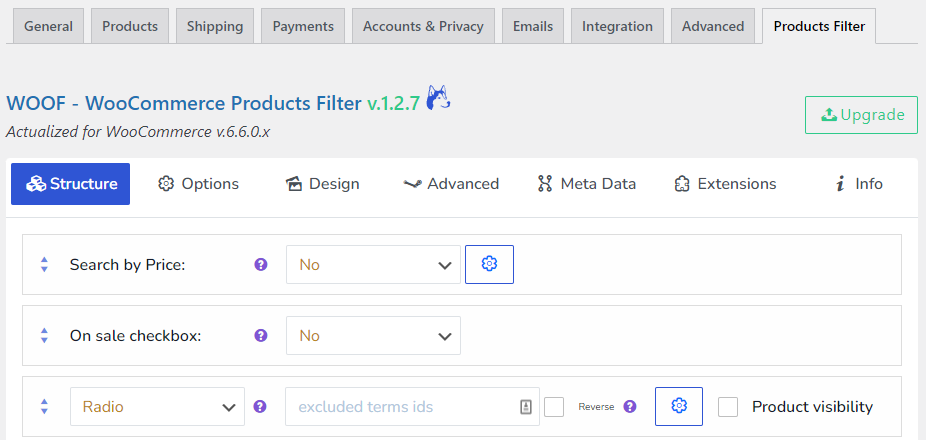This screenshot captures a detailed view of a webpage interface, specifically focusing on the "Products Filters" section of a WooCommerce-themed setup. 

At the top of the page, a series of tabs are visible: `General`, `Products`, `Shipping`, `Payments`, `Accounts and Privacy`, `Emails`, `Integration`, `Advanced`, and `Products Filters`, with the last tab highlighted.

Below these tabs, a gray bar is present, featuring on the left the title `WOOF – WooCommerce Products Filter` in blue text, followed by `V.1.2.7` in green. An icon of a wolf's head facing right is situated next to this text. Adjacent to the wolf icon is a gray bar with a green border containing the word `Upgrade` in green, accompanied by a left bracket symbol lying down with an arrow pointing upwards.

Below this, the text `Actualized for WooCommerce V.6.6.0.X` is displayed. Immediately under this are several tabs, including `Structure`, which is highlighted with a blue background, followed by `Options`, `Design`, `Advanced`, `Metadata`, `Extensions`, and `Info` in black text.

Further down, there are three distinct rows for various filtering options:

1. **Search by Price**: Featuring up and down triangles, a purple question mark, a highlighted "No" with a dropdown caret for selecting "Yes" or "No," and a settings icon on the right.
2. **On Sale Checkbox**: Displaying similar selection options as the price filter.
3. **Radio Filter**: With similar selection choices, accompanied on the far right by an option labeled `Product Visibility`, which includes a checkbox for enabling or disabling this feature.

This intricate layout provides a comprehensive overview of the customizable filter options available within the WooCommerce interface.